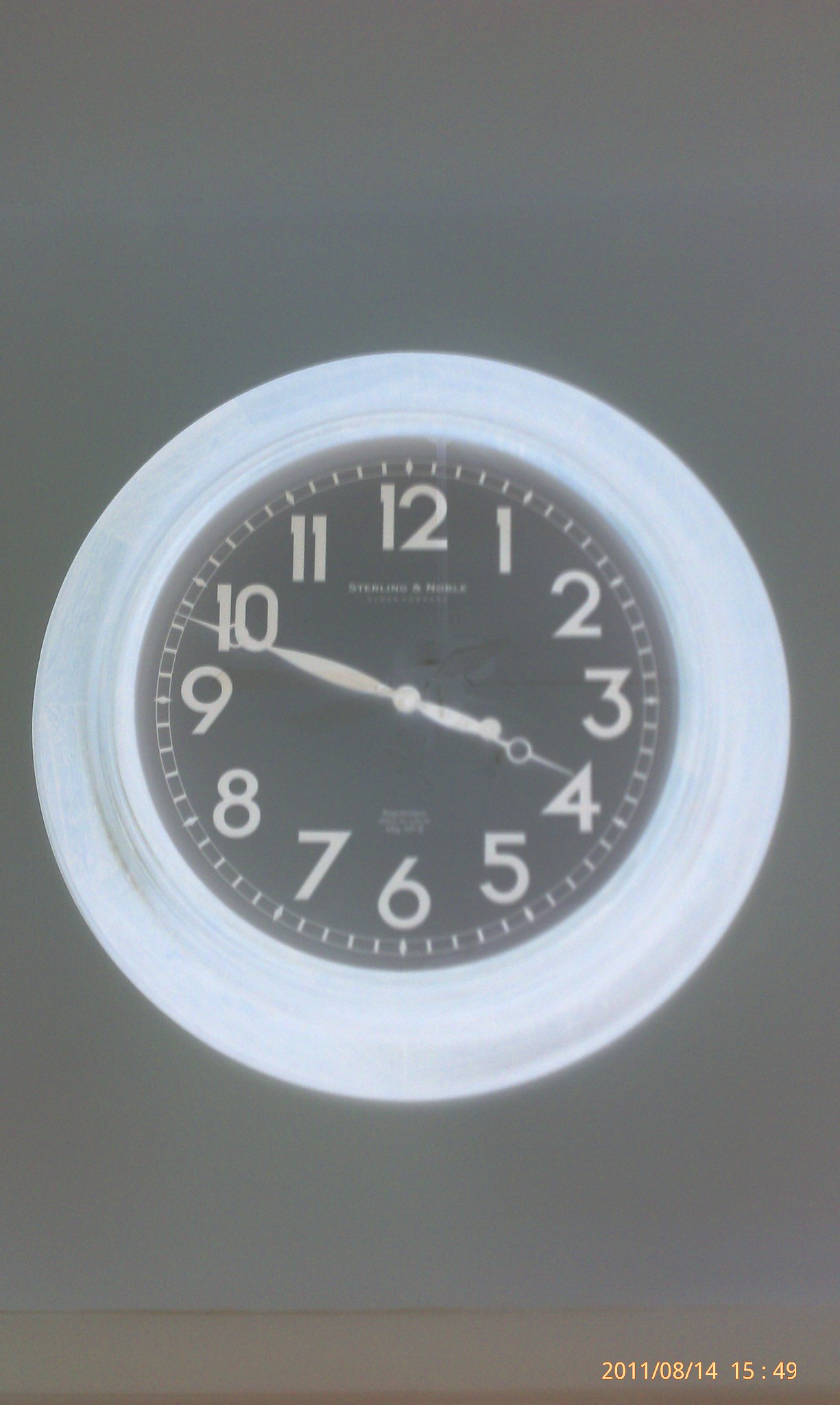This photograph features a white-rimmed clock hanging on a dark gray wall. The clock face is black with white numbers, minute markers, and hands for the hour, minute, and second. The time displayed is approximately 9:52:20. Below the number 12 is the partially legible brand name "Sterling," with another unreadable word following it. Additional indistinct writing is present above the number 6. A light brown strip at the bottom of the image includes a red timestamp reading "2011-08-14 15:49."